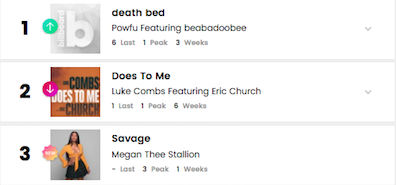The image is set against a white background and features three vertically arranged horizontal boxes outlined in a very light gray. Each box is numbered on the far left in black text. 

1. The first box, labeled as number 1, includes a gray rectangle with a bold white lowercase 'b' followed by the text "Billboard" running alongside it. To the right, in black text, the title "Deathbed" is displayed, with "POWFU" written underneath in gray, followed by "featuring B-B-Doobie." 

2. The second box, labeled as number 2, lists the title "Does to Me" in black text. Below it, the artists' names are shown in gray text: "Luke Combs featuring Eric Church." Additionally, there is an image associated with this entry that features the word "Combs" in black text, "Does to Me" in white text overlaid on top, and "Church" in black text at the bottom.

3. The third box, labeled as number 3, indicates the title "Savage" in black text, followed by "Megan Thee Stallion" in gray text below. An associated image showcases Megan Thee Stallion standing and wearing an orange top paired with a black miniskirt.

Each box is consistently outlined in light gray, maintaining a clean and organized appearance.